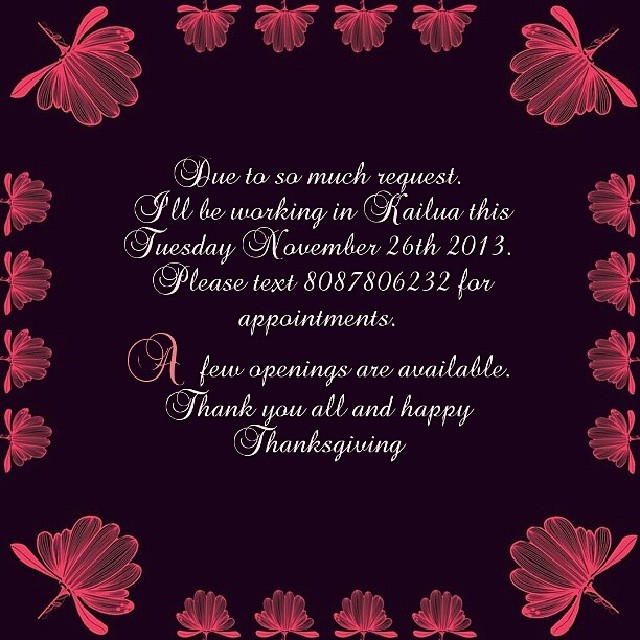This square-shaped invitation features a dark background, possibly black or deep brown, adorned with an intricate floral border. Large pinkish-red flowers are prominently displayed in each of the four corners, with smaller, matching flowers filling in the spaces along the sides. The invitation text is written in flowing cursive, predominantly in white, except for the word "a," which is highlighted in a pinkish hue that echoes the color of the flowers. The central message reads: "Due to so much request, I'll be working in Raylua this Tuesday, November 26, 2013. Please text 808-780-6232 for appointments. A few openings are available. Thank you all and Happy Thanksgiving." This elegant and detailed notification appears to be intended for clients, informing them of a special work schedule due to high demand.